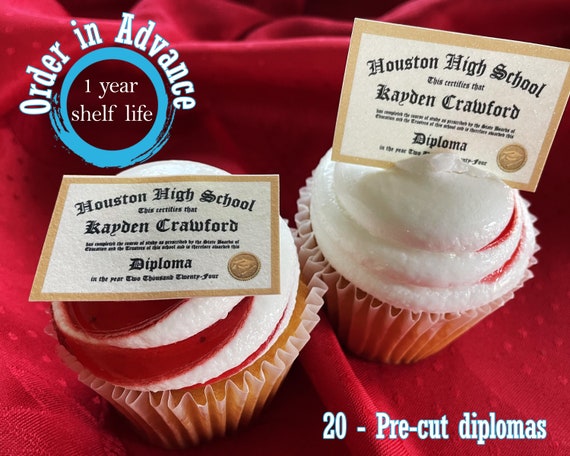The image is a detailed advertisement for a bakery product, specifically cupcakes designed for graduation parties. In the top left corner, the text reads "Order in advance, one year shelf life," highlighted by a blue circle. The bottom right corner features the text "20 pre-cut diplomas," indicating that the product includes twenty edible, pre-cut diplomas.

The main focus of the image is two cupcakes placed side by side on a red fabric background. The cupcakes are adorned with white frosting swirled with red. Each cupcake is topped with a miniature edible high school diploma. The diplomas are detailed, displaying "Houston High School" and the name "Caden Crawford," with the word "diploma" prominently visible at the bottom of each diploma. The image is bright and clear, benefiting from natural light, and effectively showcases the product aimed at celebrating high school graduations.